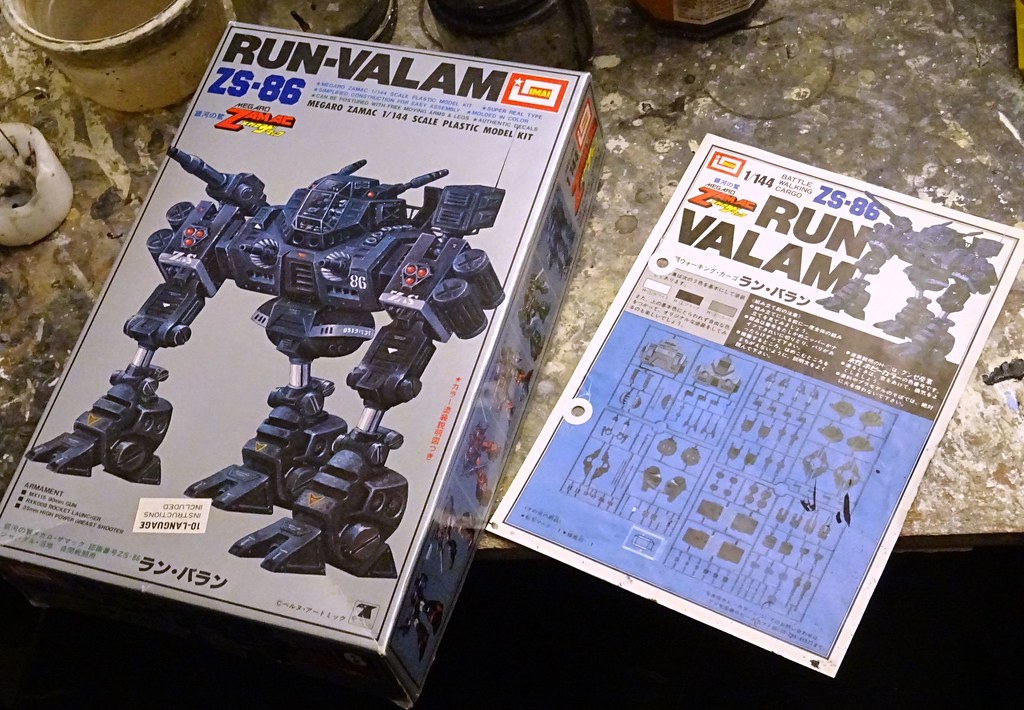This image features a detailed toy robot model kit displayed prominently on a brown-gray countertop. On the left, there is a gray box with the title "Run-Valam, ZS-86" on the top, and the description "Megaro Zamac 1/144 scale plastic model kit" beneath it. The box showcases an image of a complex, dark gray and black robot with three hydro-pressure air legs—two in the front and one in the back. The robot's design includes a cockpit in the head where miniature figures can presumably sit and operate the machine. Beside the box on the right is a one-page instruction brochure, which also features an image of the robot. The brochure is titled "Run-Valam" and provides a diagram displaying all the parts included in the kit. Both the box and the instruction sheet contain writing, much of which is in Japanese, indicating the model's intricate and likely foreign origin. The items are neatly arranged next to each other, emphasizing the kit's comprehensive nature.